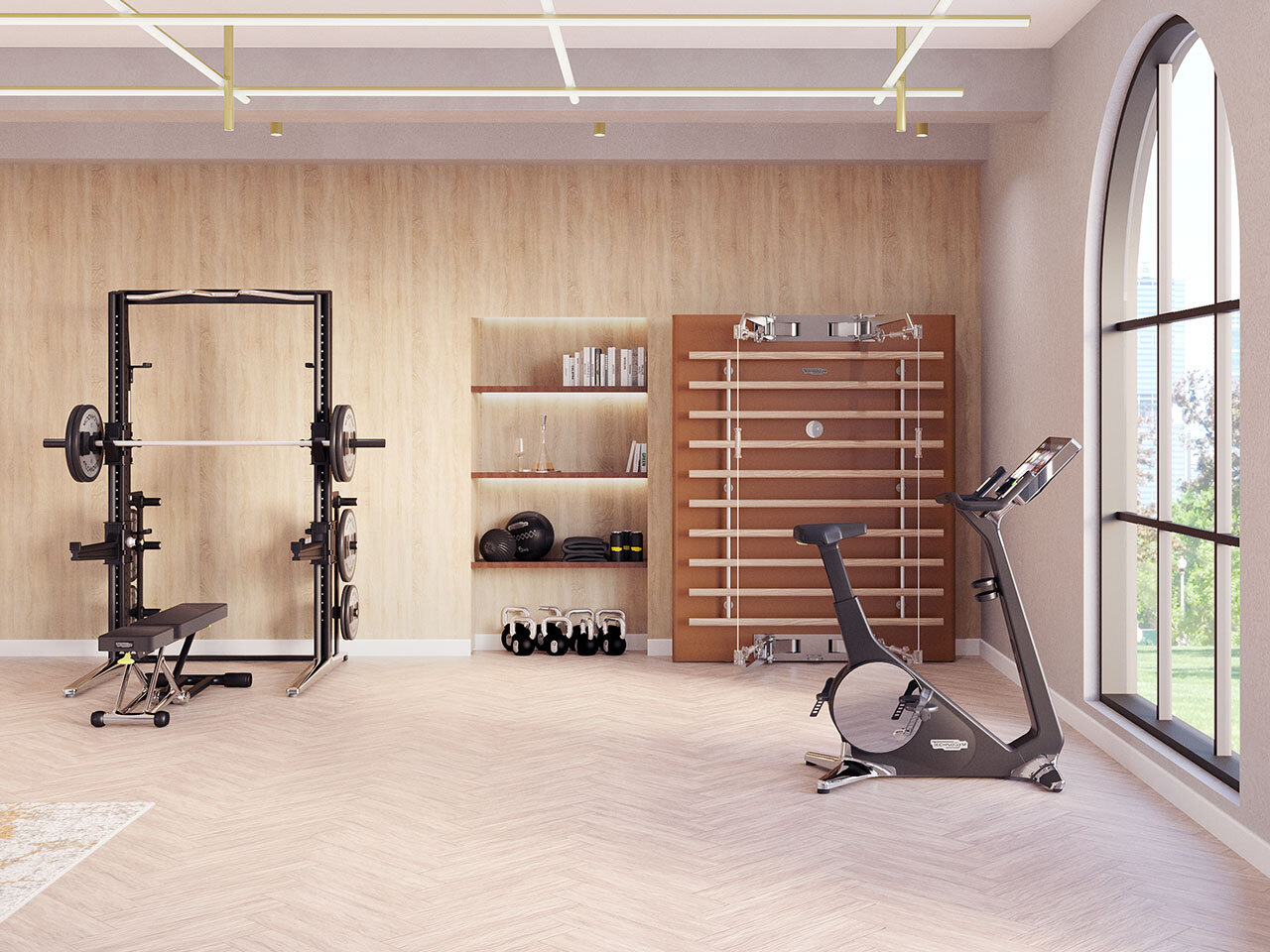The image showcases a spacious and professionally equipped home gym with a neutral palette, featuring off-white wavy tile floors interlaid with a subtle zigzag wood pattern. Centrally positioned is a weight bench adjacent to an iron stand equipped for pull-ups and holding racks of various weights. To the right, an arched window with black panes offers a view of trees outside, flooding the space with natural light. In front of the window sits a sleek black, white, and gray stationary bike equipped with a screen for virtual rides. Beneath the window, kettlebells are neatly arranged on the floor. On the right wall, an inset bookcase houses an eclectic mix of books, workout equipment, candle holders, and what appear to be bowling balls on the shelves. Above, suspended from the ceiling, are rectangular bars in white and gold, enhancing the room's modern aesthetic. An area rug in a light beige hue marks the lower left corner of the room, adding a cozy touch to this well-appointed exercise space.